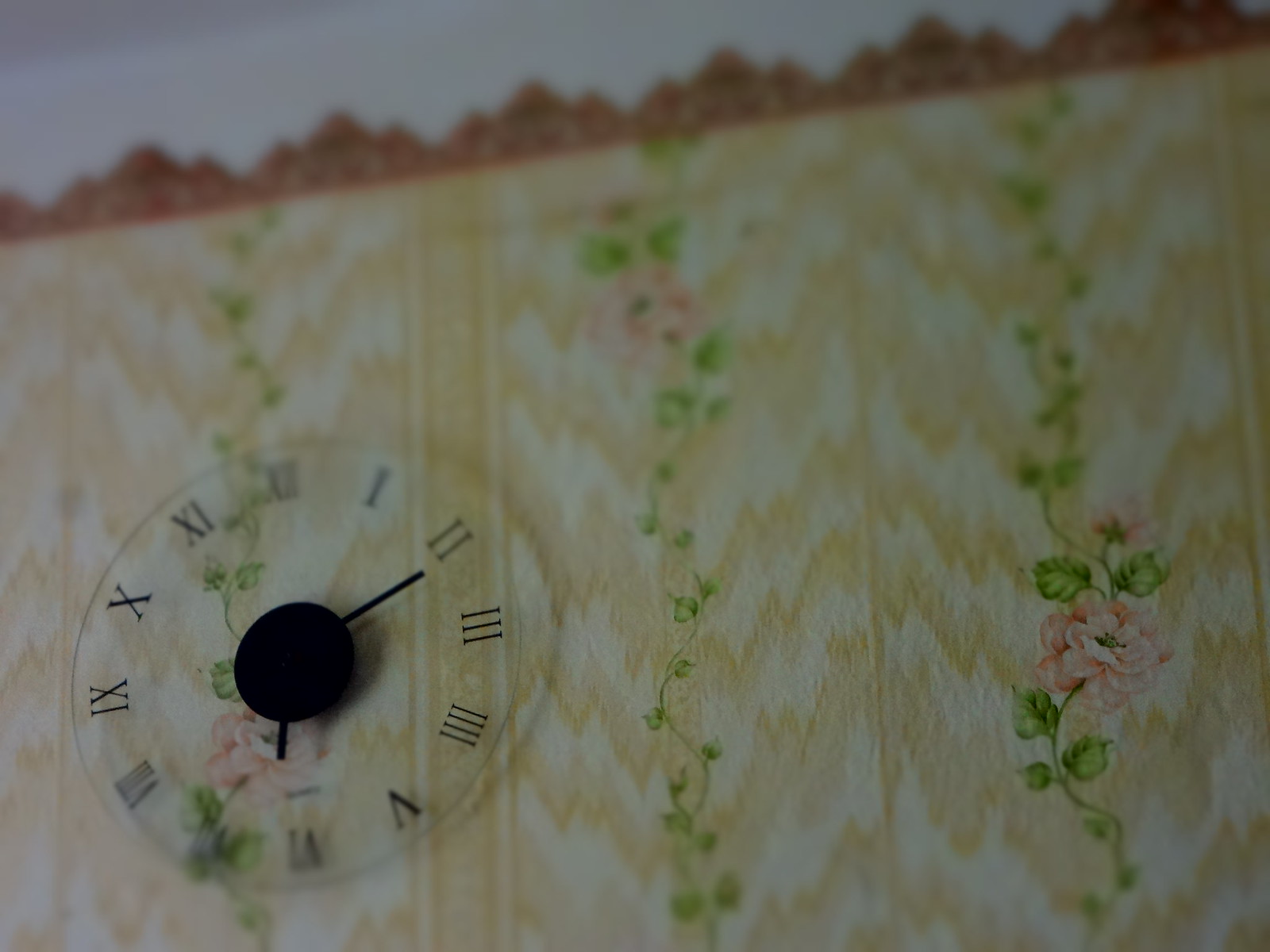This photograph captures an elegant, decorative-style clock prominently featured against a vibrant background. The clock itself has a circular, translucent face, with black Roman numerals from I to XII marking the hours. Absent of any minute markers, the minimalist design is accentuated by a sleek, black, circular button in the center, from which the black hour and minute hands extend. The time displayed is approximately 6:12. The backdrop is a visually engaging fabric-like design, showcasing a zigzag pattern in white and yellow. This vibrant pattern is adorned with cascading green vines interspersed with delicate pink roses, adding an element of natural beauty to the composition. The top corner of the image includes a small portion of a white background wall, emphasizing the focus on the ornate clock and its colorful setting.